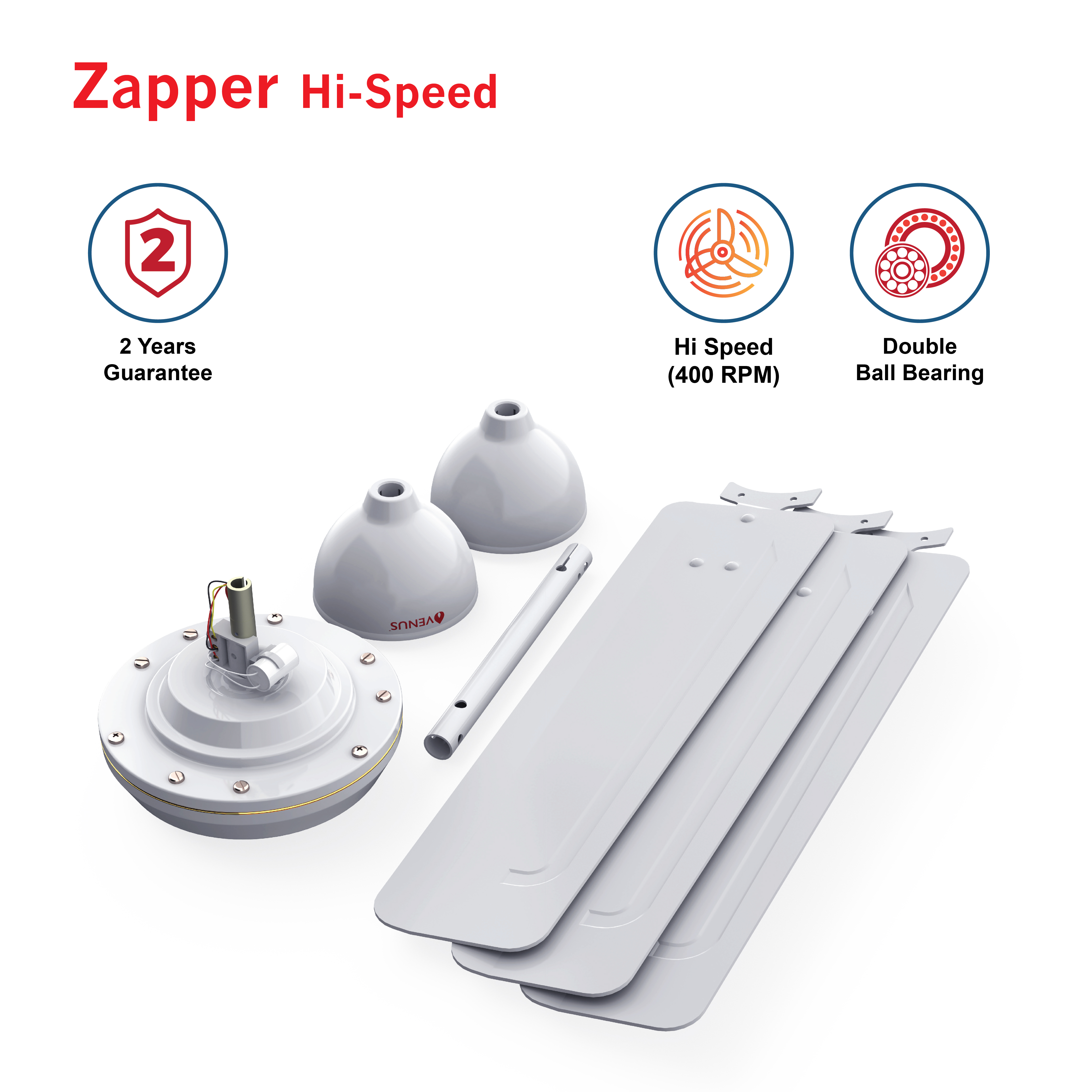The image is a detailed product advertisement set against a white background, likely for a manufacturing component. In the upper left corner, the product name "Zapper High-Speed" is prominently displayed in red font. Below that, a series of three blue circles with white backgrounds provide further details: the first circle features a red shield with the number "2" inside it, followed by black text that reads "Two years guarantee". The second circle contains an image of an orange fan with the caption "High-Speed, 400 RPM" in black text below it. The third circle shows two red ball bearings side by side, with the caption "Double Ball Bearing" in black text underneath. 

The product itself, predominantly white or light gray, includes several components: a large circular part that appears to be a ball bearing with silver bolts, two conical parts resembling lamp shades with holes at the top, a cylindrical metal rod with two black holes, and three long, rectangular fan blades with rounded corners stacked together. The fan blades are a shade of off-white. This intricate layout of parts implies that the product is composed of various interconnected components, possibly for a high-speed mechanical function.